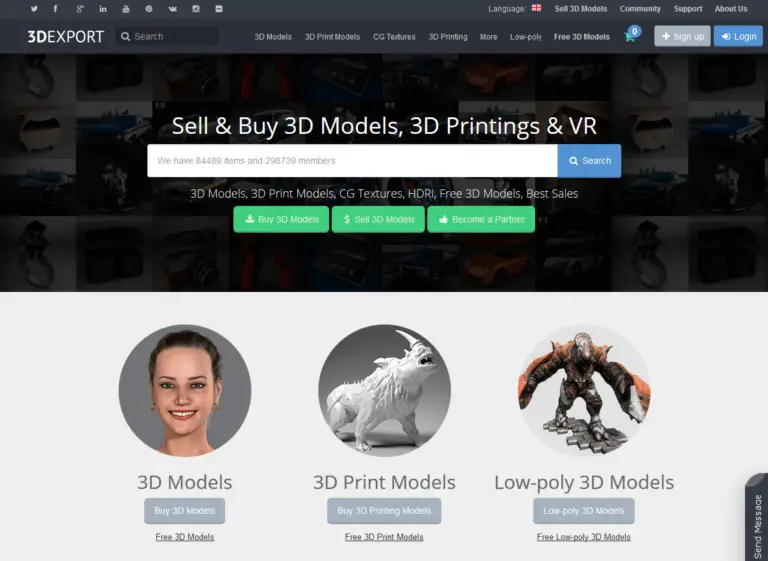The image depicts a computer screen displaying a website interface on either a Windows or Mac computer. The layout appears slightly wider than tall. The top half of the screen features a sleek black background, while the bottom half is contrasted in off-white.

At the very top right corner, there are several small, indistinguishable icons, approximately eight in total, arranged horizontally. Moving towards the top left, there's a language indicator, resembling an English flag, followed by menu options such as 3D Models, Community Support, and About Us.

Below these elements, prominently displayed in large font, is the text "3D Export." Directly beneath this title, a search bar is accompanied by several small, selectable tabs offering various options. Further right, the interface includes a shopping cart icon, a Sign-On button, a Sign-Up button in gray, and a Log-In button in blue.

Centered on the page, a bold message reads "Sell and Buy 3D Models, 3D Printers, and VR," followed by a white input bar to enter text, flanked by a large blue button. Underneath, faint text is noticeable, along with three small green buttons with various download options.

The lower off-white section of the page is neatly divided into three columns. The left column highlights "3D Models," illustrated by a circular image of a computer-generated woman above a gray button. The middle column showcases a "3D Print Model," depicted with an image of a mythical creature in a similar circular frame, also accompanied by a gray button. The right column features "Low Poly 3D Models," typified by a griffin-like creature and includes a gray button as well.

This cohesive design emphasizes user engagement through intuitive navigation and clear call-to-action elements, catering to enthusiasts and professionals in the 3D modeling, printing, and VR realms.